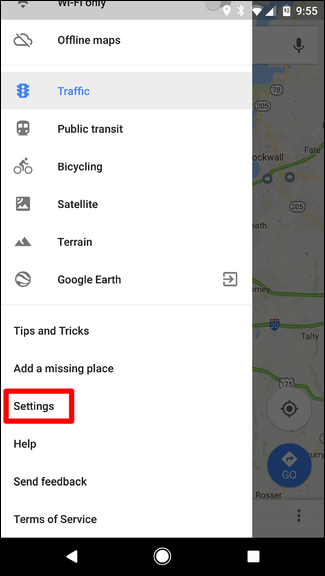The image depicts a smartphone screen displaying a partially covered map application. From the left side, a white menu has popped up, obscuring most of the screen except for a slim vertical strip on the right. The map underneath appears to have vibrant colors muted by a grayish overlay.

At the top of the screen, various status icons are visible, including Bluetooth, Wi-Fi, cellular signal strength, and a battery level at 92%. The time displayed is 9:55. 

The top segment of the white menu shows the text "Wi-Fi only," partially cut off. Below this, various options are listed: "Offline maps," "Traffic" (highlighted in blue), "Public transit," "Bicycling," "Satellite," "Terrain," "Google Earth," "Tips and tricks," "Add a missing place," "Settings" (highlighted with a thick red rectangle, seemingly added post-production), "Help," "Send feedback," and "Terms of service."

At the very bottom of the screen, a black strip features three white navigation icons: a left arrow (back button), a circle, and a square.

The overall context suggests that this image is intended for educational purposes, demonstrating how to navigate the settings for viewing traffic within the map application.